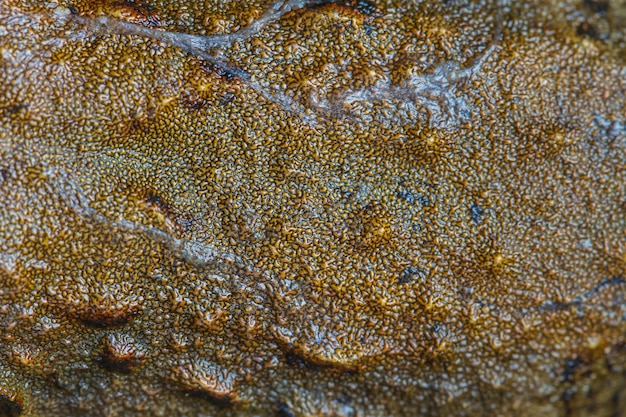In this photograph, a highly detailed, slimy, and bumpy texture is showcased, likely depicting an organic surface found in nature. The primary colors blend in shades of yellowish-brown, gold, and beige, creating an earthy palette. Interspersed throughout are veins of slime and dark brown or black markings, resembling trails left by slugs or other creatures. The surface is not smooth; instead, it is raised and lumpy, adding to the visual complexity. Small black flecks are scattered across, and some areas are tinged with green, potentially hinting at algae or plant matter. The texture and coloration are reminiscent of a toad's skin or a slimy rock submerged in water. Gray and black strands weave through the scene like veins, giving it an almost coral-like appearance. Overall, the image captures a wet, glistening, and organic material that feels both intriguing and slightly repulsive, possibly representing a natural object or an artistic recreation with no clear context.